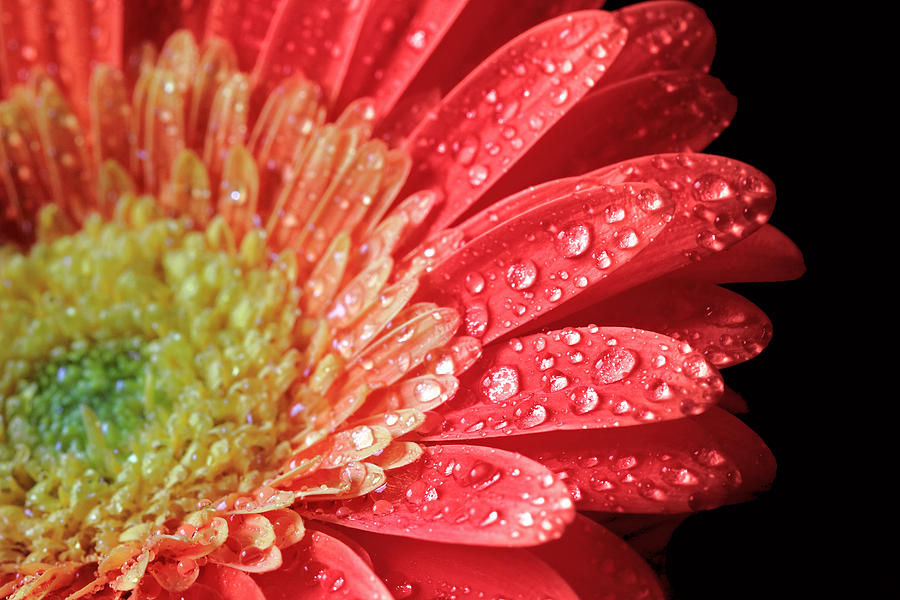This is a close-up rectangular photograph, approximately five to six inches wide and four inches high, that showcases the intricate details of a flower against a black background. The flower is positioned from the left-hand side, extending about four-fifths of the way across the image, and slightly offset toward the bottom left. The center of the flower features a rounded, flat stamen with a light green in the very core and surrounded by yellow. The petals are numerous and layered; starting with short and narrow light yellow ones near the center, transitioning to lighter pink, and finally becoming long, elliptical, and bright pink towards the outer edges. There are about six or seven rows of petals in total. The entire flower is misted with water droplets of various sizes, resting on both the outer and inner petals, enhancing the textured, delicate quality of the image. The sharp contrast with the black background accentuates the vibrant colors and details of the flower.